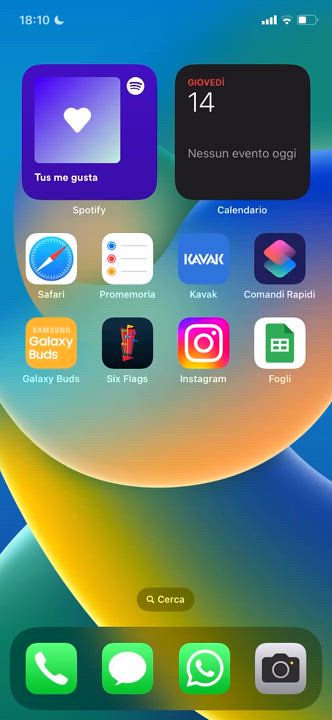This detailed caption accompanies a screenshot of a phone screen. 

The time is displayed in military format at the top of the screen, reading 18:10, which translates to 6:10 PM. On the top right corner, the phone's internet connection is indicated by a signal strength icon resembling a staircase, with all the bars fully filled in white, signifying a strong connection. Next to it is the battery icon showing that the battery is less than half charged, as the white fill inside the battery outline is below the halfway mark.

On the upper left part of the screen, a Spotify notification shows the song "Tu Me Gusta" currently playing, accompanied by the Spotify logo consisting of three horizontal lines stacked vertically, resembling air conditioning vents. Additionally, on the top right, the date is displayed in the format "Giovede 14," likely indicating Thursday the 14th, encased in a black square.

Moving downward, the first row of app icons, from left to right, includes Safari, Pro Memoria, Cavac, and Comandi Rapidi. The following row features icons for Galaxy Buds, Six Flags, Instagram, and an app labeled Fogly, which appears to be Google Sheets.